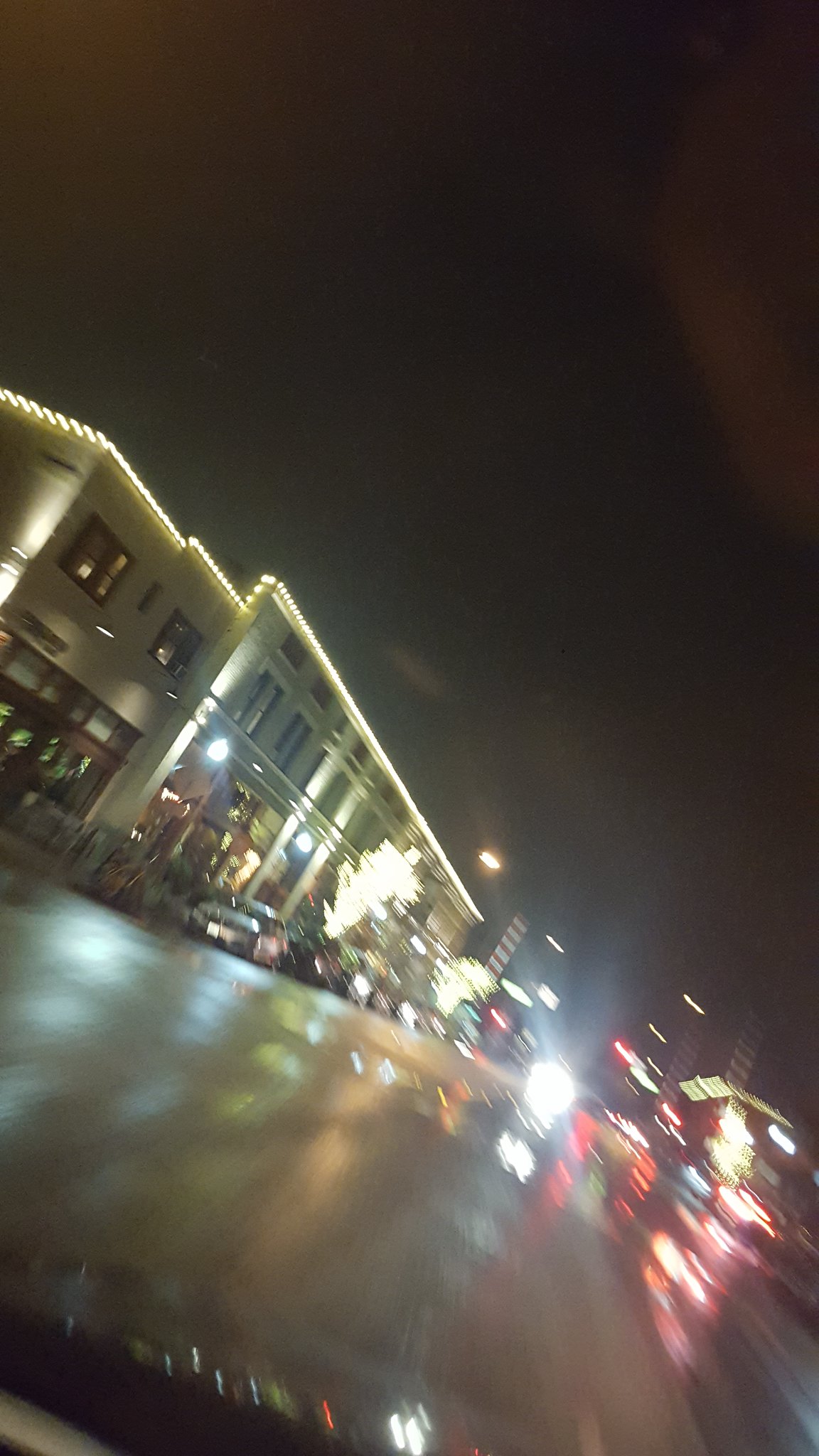This photograph, taken from inside a moving car, captures a nighttime street scene through a slightly diagonal windshield, angled downward to the right. The blurred image shows a wet road running from mid-left to bottom-right, reflecting the white lights of the surrounding environment. Prominently to the left, there is a long, two-story tan building adorned with white lights along its rooftop. Attached to it is a smaller, square structure. Both buildings feature windows on the first and second stories, possibly indicating stores below and apartments above. In front of these buildings are a couple of parked cars and light-adorned trees. The oncoming headlights of a distant car are visible through the blurred streaks of light, adding to the dynamic, yet slightly disoriented feel of the image. The night sky above looms dark and uninterrupted.